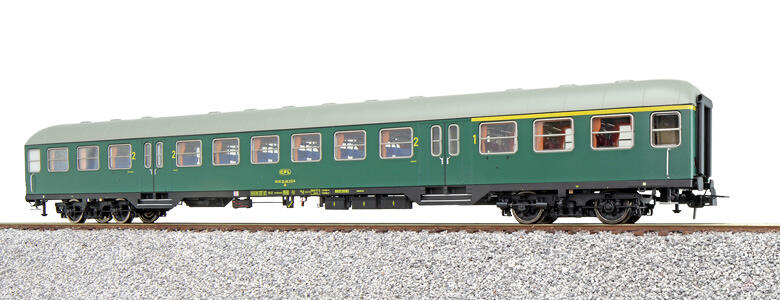This color photograph depicts a highly detailed close-up of a long, green train car positioned slightly diagonal and pointed towards the right. The train is situated on a small brown track, which rests on gray-white gravel. The entire backdrop is stark white, highlighting the train car as the main focus of the image; this composition gives the impression that it could be an advertisement for a model or toy train due to its immaculate presentation.

The train car itself is a rich, dark green with a lighter green or white roof, adorned with numerous windows that feature salmon or orangey curtains. These curtains are all open, allowing a glimpse through to the other side of the car, although no passengers are visible. Notable details include black wheels beneath the car and various markings and numbers in yellow, with a prominent '2' repeated along the side. There is also a distinct yellow stripe at the front end of the car, further designating its orientation. The overall image is wider than it is tall, capturing the complete essence of this classic, isolated passenger train car.